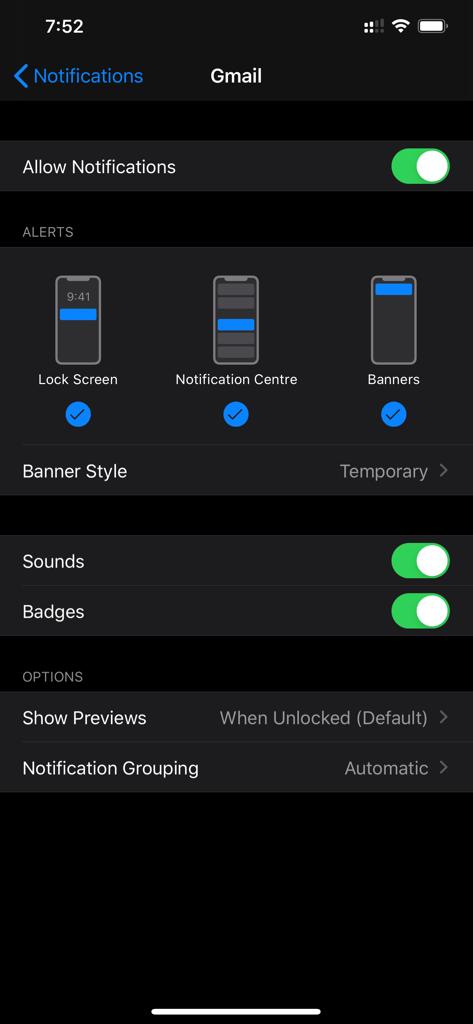The image displays a phone screen with a black background. In the top left corner, the time "7:52" is shown in white font. To the right, there are icons for Wi-Fi, signal strength, and battery status. Below, a notification is visible with a blue arrow pointing left and "Gmail" in white font at the center. Beneath, in a gray circle, it reads "Allow Notifications" in white font. The toggle button is turned on, outlined in green.

Further down, on a black background, "Alerts" is written in gray font to the left. Below this, in a lighter gray box, there are three phone icons labeled "Lock Screen," "Notification Center," and "Banners," each with corresponding gray check marks in blue circles underneath. The "Lock Screen" icon displays the time "9:41" within a blue screen. The "Banners" icon has a blue highlight at the top, while the "Notification Center" icon features a gray highlight in the middle.

Below these icons, "Banner Style" is labeled in white font to the left, with "Temporary" indicated in gray font to the right, followed by an arrow pointing right. Further down, options for "Sounds" and "Badges" are displayed with toggles turned on, indicated by white circles. Additional options include "Show Previews" set to "When Unlocked" (default) with a gray arrow, followed by "Notification Grouping" labeled "Automatic" in gray font, also accompanied by a gray arrow. At the very bottom, a thick white line spans the screen.